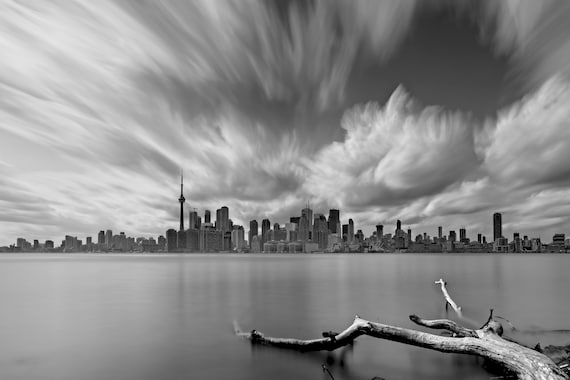In this striking black-and-white photograph, the viewer's eye is drawn to a sprawling cityscape dominating the midsection of the image, defined by numerous towering skyscrapers and a distinctive needle-like structure jutting into the sky. The top half of the image features wispy, stretched-out clouds that appear to be in motion, suggesting this might be a frame from a time-lapse video. The smooth expanse of a vast, gray-toned body of water covers most of the lower portion of the photograph, with a dead tree branch breaking the uniformity in the lower right corner. This log, with its intricate branching, adds a touch of natural elegance to the otherwise urban composition. The overall scene, viewed from a riverbank, offers a hauntingly beautiful, almost surreal atmosphere due to the blurred cloud effect from the possible lens manipulation and the stark monochromatic palette.